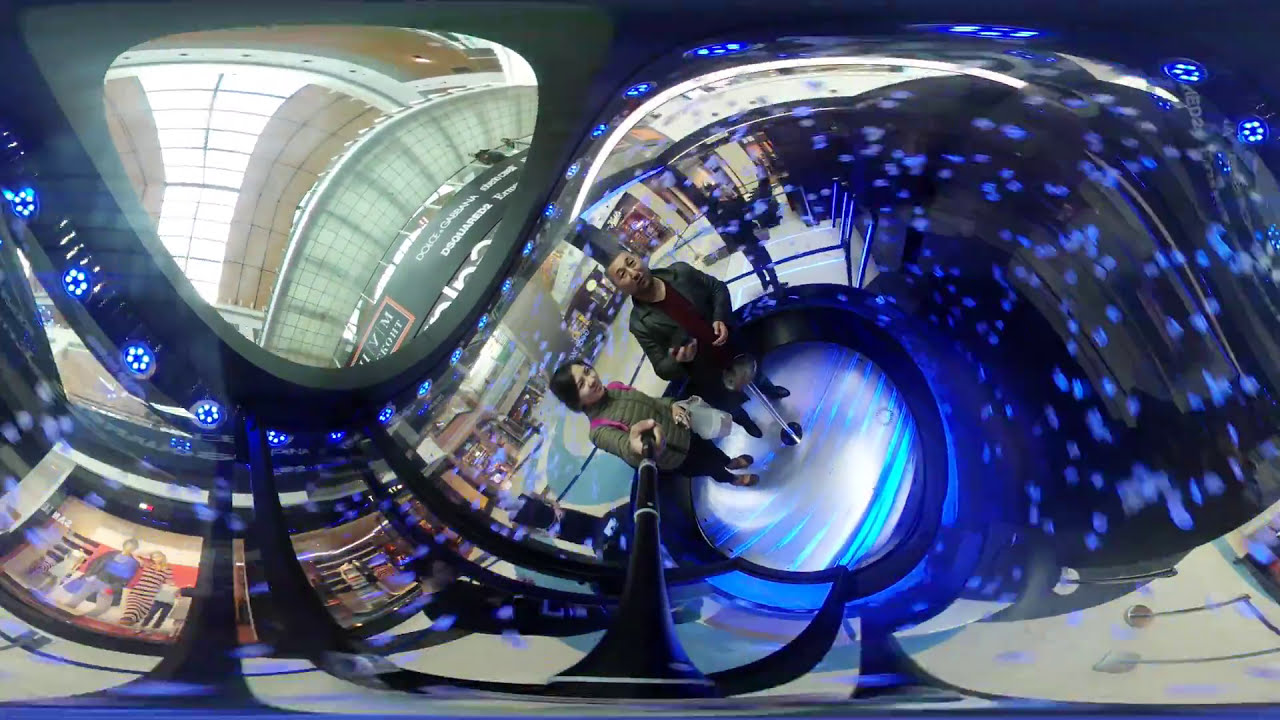In this image, two people stand inside a glass-encased space simulator located in a mall. The young woman on the left, dressed in a green, puffy winter jacket and holding a selfie stick, appears to be in her 20s. Posed beside her is an older man in his 40s, wearing a black leather jacket over a maroon shirt. Both are looking up at the camera. The space behind them is illuminated by numerous blue lights, mimicking the appearance of outer space. The image is notably distorted, with the scenery appearing twisted and curved, giving the photo a surreal, panorama-like effect. Through the enclosure, you can glimpse the mall’s interior, including various stores on the left with one sign reading "Dolce and Gabbana" and another partially visible sign. The photo's warped nature creates an almost dreamlike, whimsical atmosphere, particularly emphasized by the sparkles surrounding the simulator.